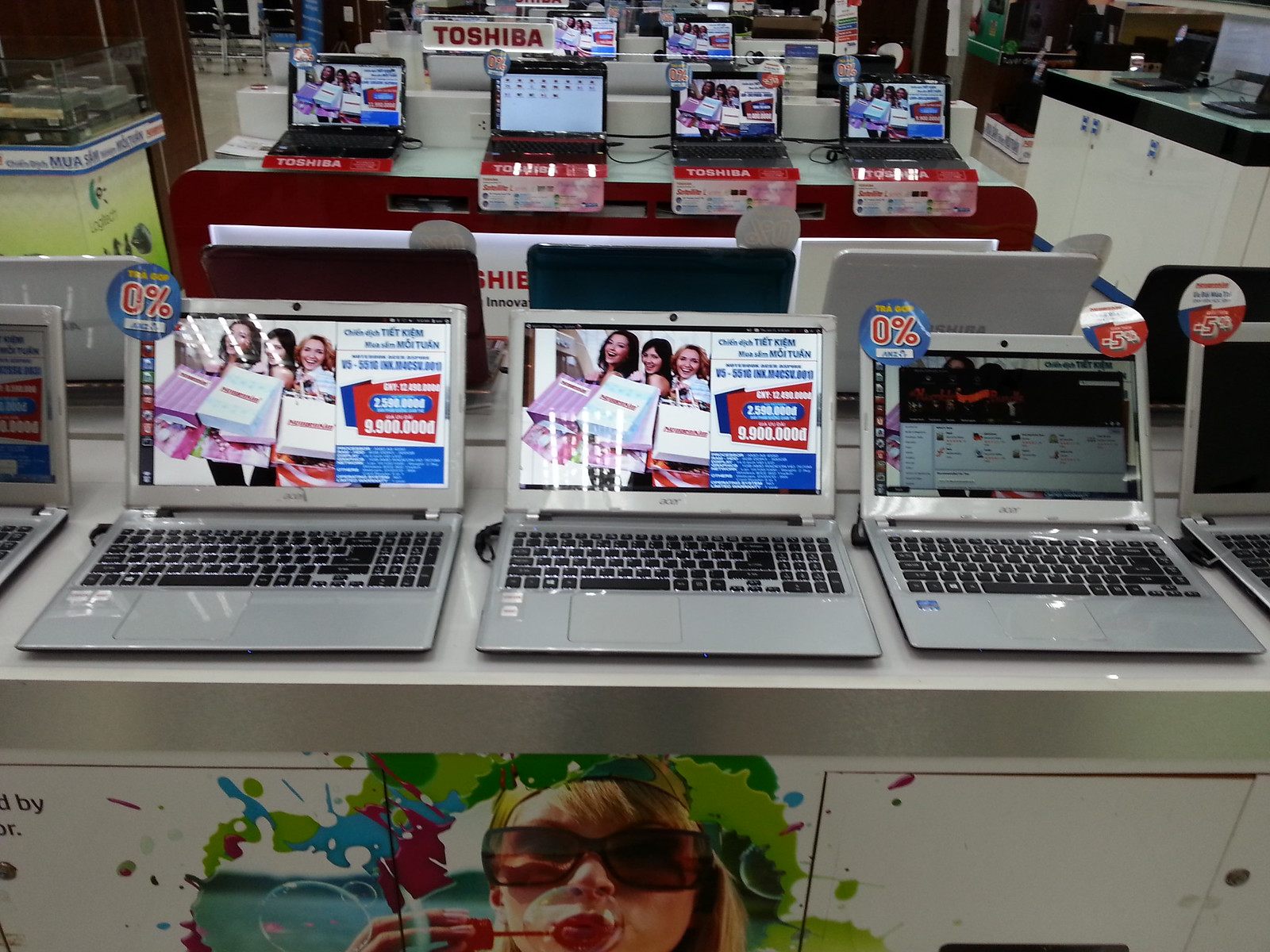The photo captures an electronics store teeming with various laptop displays. At the forefront, a table showcases Acer laptops that are silver with black keys. Two of these laptops present advertisements featuring three women, possibly Vietnamese, holding multiple shopping bags. One laptop’s screen has stickers indicating "0%" and "5%." This front display table is adorned with a colorful decor that includes splashes of green, red, and blue paint and features an illustration of a blonde woman with sunglasses blowing bubbles, donning a hat. Moving to the background, we observe another row of laptops, primarily Toshibas that are black, situated on cream-colored countertops. Signs prominently display the Toshiba brand in red letters alongside promotional material indicating various discounts like "0%" and "-5%." The entire setup exudes the vibrant yet functional atmosphere typical of a bustling electronics store, with laptops in different rows and layouts methodically arranged for customer viewing.